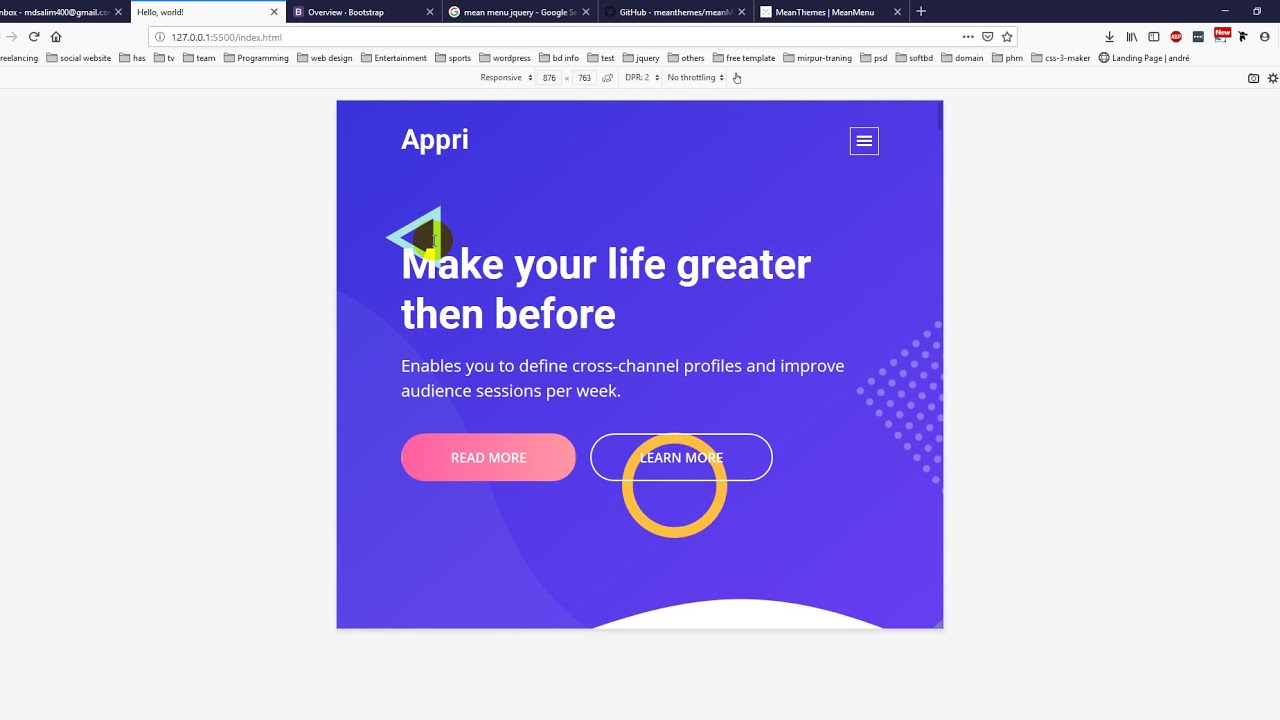The image is a screenshot of a web page with a primarily white background. This is the second tab out of six different tabs, and it is the active one. The highlighted tab displays a large, blue, square-like image. In the top-left corner of this square, the name "Apri" is written in white letters. Opposite this, in the top-right corner, there is an icon consisting of three horizontal lines inside a square, suggesting it might be a settings or details button.

Dominating the main section of the blue square is the slogan, "Make your life greater than before." Below this slogan, there is a brief description stating, "It enables you to define cross-channel profiles and improve audience sessions per week."

Toward the bottom of the blue square are two buttons. The first button is pink and prominently highlighted, with the text "Read More" in white. Next to this, there is a blank horizontal button with the words "Learn More" in white, superimposed over a round yellow circle illustrated on the blue square.

The blue square itself features a couple of geometric patterns: a triangular arrangement of dots in a grid pattern on one side and a light blue wavy area on the other. Completing the design at the bottom of the square is a small, white arc with a line beneath it, following the curvature upwards and aligned with the square's perimeter.